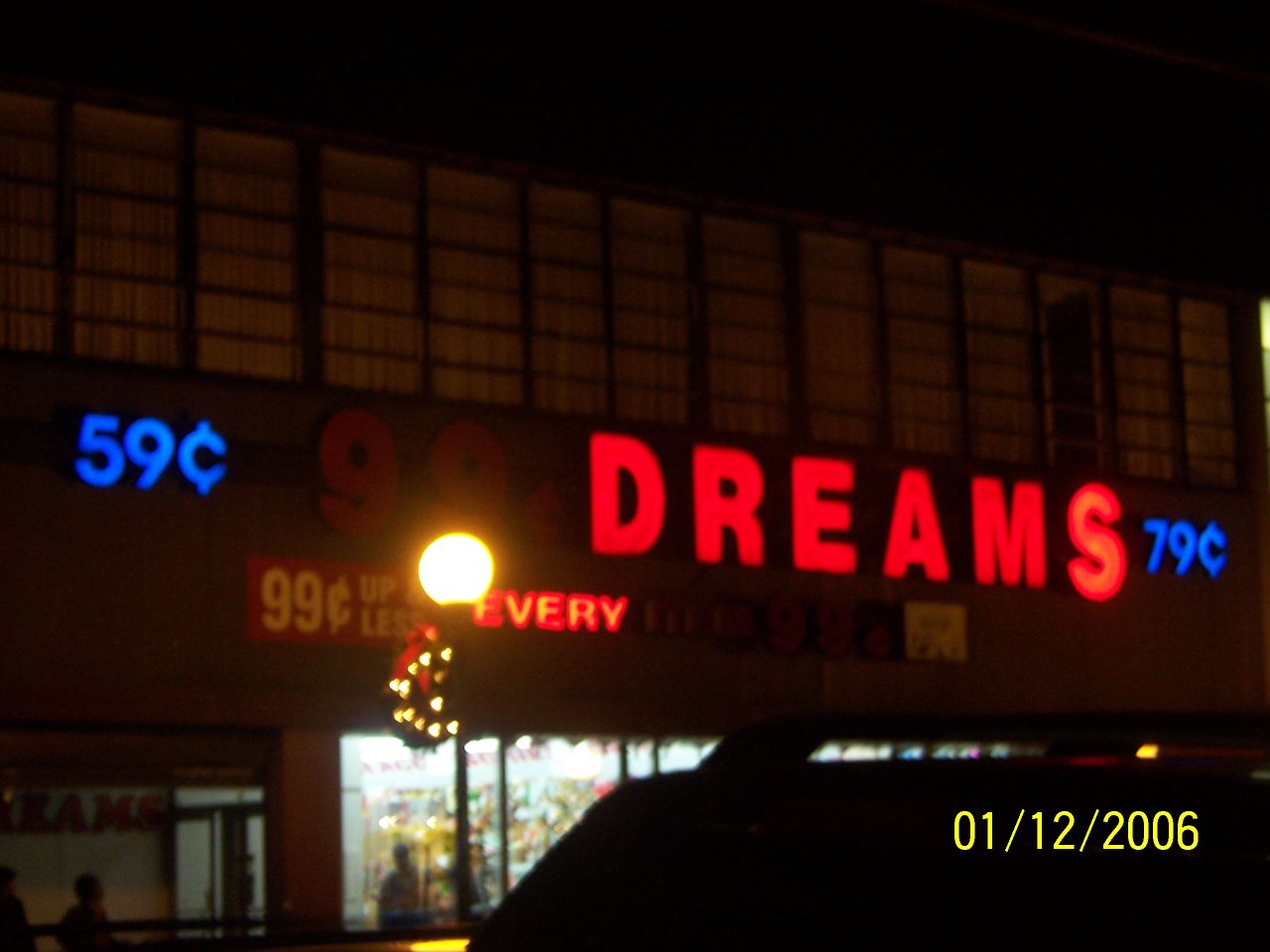Captured on January 12, 2006, this nighttime photograph showcases the exterior of a store. The absence of flash leaves the surrounding environment cloaked in darkness, emphasizing a vivid neon sign as the focal point. This neon sign, sprawling across the middle of the image, features massive text with varying colors and messages. On the left, the sign displays "59 cents" in blue, transitions to "99 cent dreams" in red at the center—though the "99 cent" part isn’t illuminated—and concludes with "79 cents" in blue on the right. The word "dreams" is particularly large and stands out prominently. Positioned above this central sign is a red and yellow banner proclaiming "99 cents & less." Below "99 cent dreams," another neon sign displays the word "EVERY" brightly, alongside another partially lit but discernible "99 cents." The store itself appears open and lit from within, with a person faintly visible inside. Additionally, a vehicle, likely a car or van, is parked at the bottom right corner, near the edge of the frame. The image is timestamped with the date 01/12/2006.